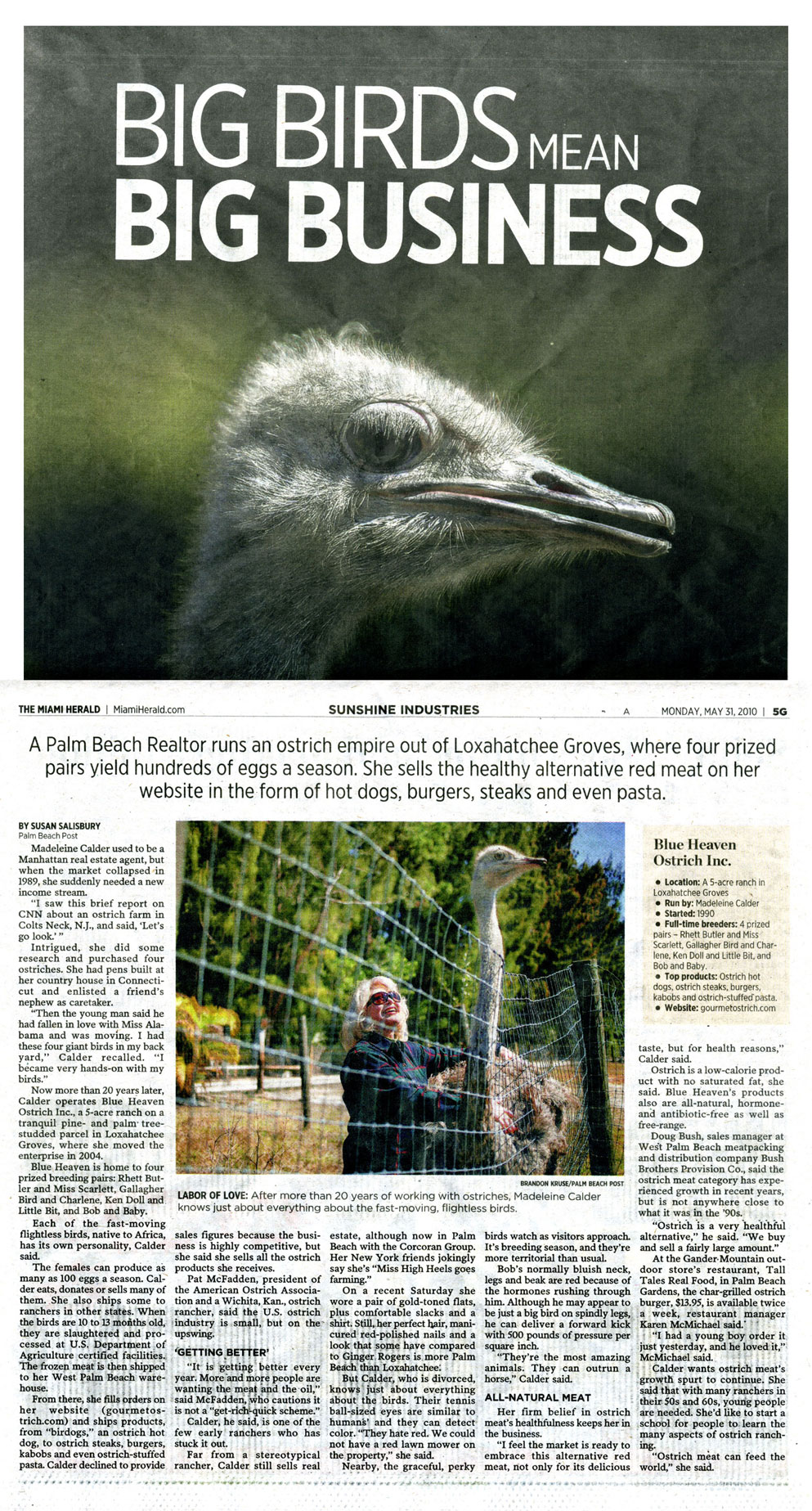A captivating article is headlined with a bold image captioned "Big Birds Mean Big Business," emphasizing the growing ostrich industry. The central photograph showcases a close-up of an ostrich's head, detailing its unique features. The intricate textures of the ostrich's feathers, which appear almost fur-like, are clearly visible. The beak, strikingly black, stands out in sharp contrast to the rest of its face. Remarkably, the ostrich's eye is captured with such detail that a subtle, greenish-black film can be observed, a feature not often noticed. 

Below, the article delves into the story of a Palm Beach realtor who has established an ostrich empire in Loxahatchee Groves. Accompanied by a photograph of the realtor with an ostrich, the caption explains that she manages to produce hundreds of eggs per season from her prized pairs. Offering a healthy alternative, she markets ostrich meat on her website, presenting it in various forms including hot dogs, burgers, steaks, and even pasta.